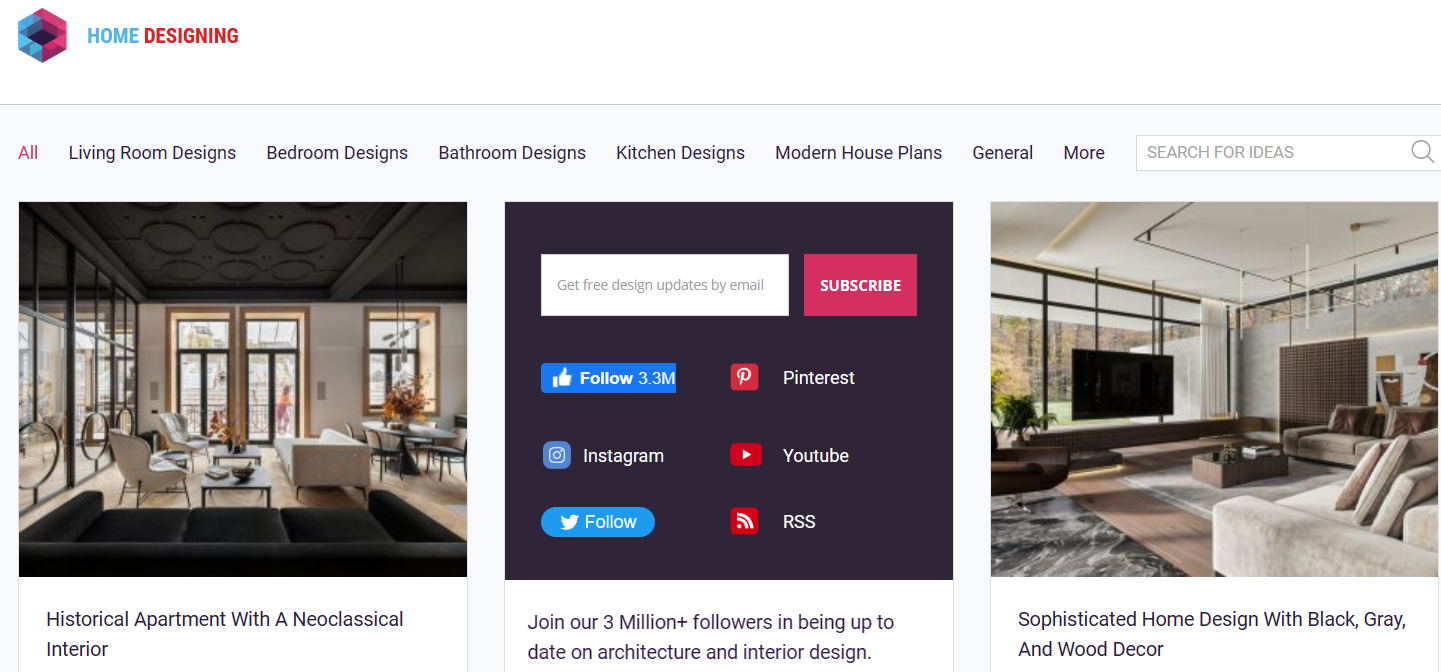The image displays a website interface with a white border at the top, featuring a hexagonal icon split into blue on the left and purple on the right. To the right of the icon, the word "Home" is written in blue, followed by "Designing" in red. Below this, the interface has a gray background with a navigation menu at the top offering various options: All, Living Room Designs, Bedroom Designs, Bathroom Designs, Kitchen Designs, Modern House Plans, General, and more. Beneath the navigation menu, there's a search box labeled "Search for Ideas" with a magnifying glass icon. Below the search box, three images are displayed. The first image, on the left, showcases a cozy living room featuring chairs and a sofa. The middle image is a subscription prompt where users can enter their email address. The rightmost image portrays another stylish room with couches, a flat-screen TV, and large, tall windows that allow for ample natural light.